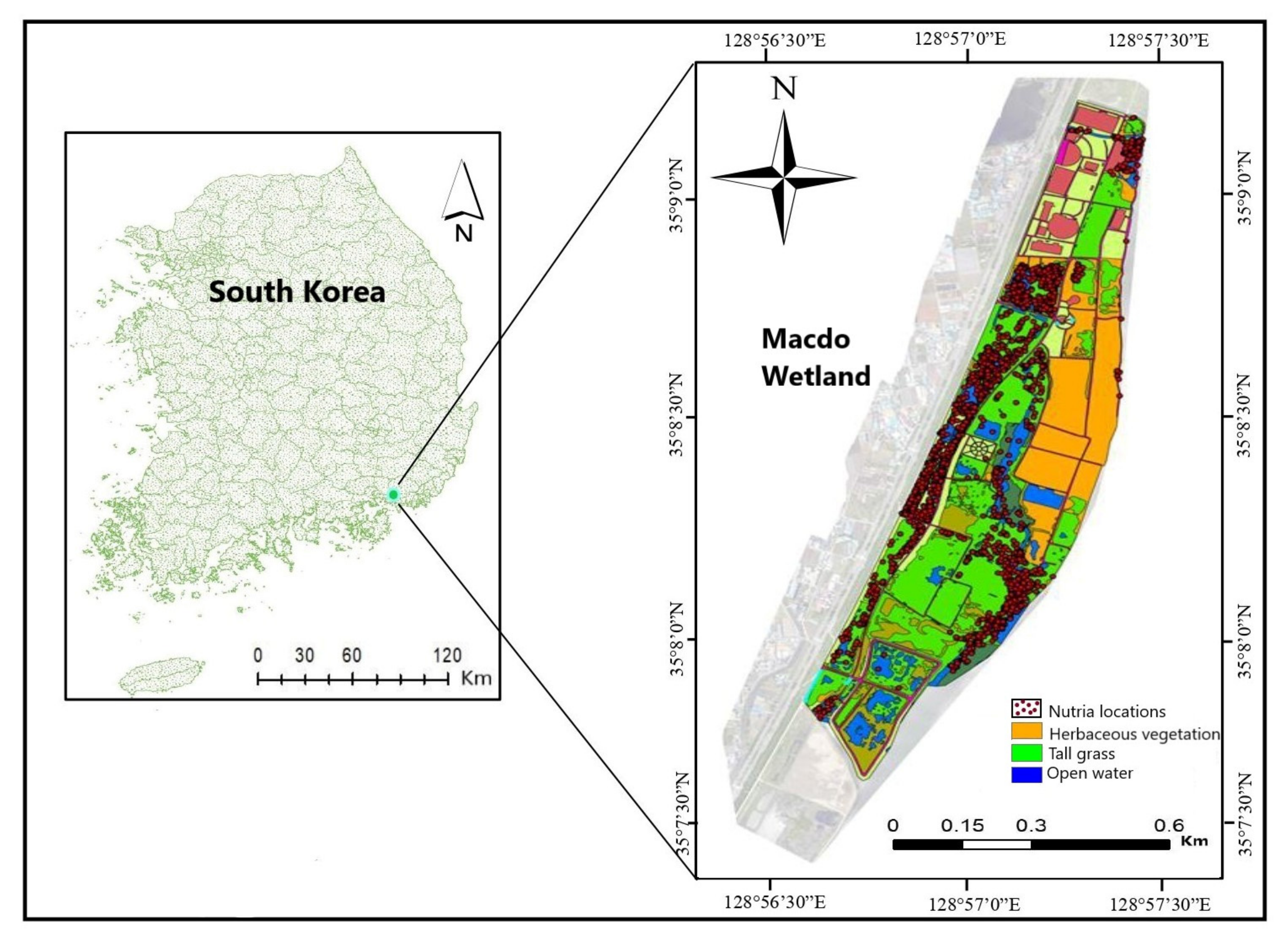The image displays a detailed map of South Korea on the left, labeled in bold black text. The map includes a north-pointing compass and a scale from 0 to 120 kilometers. A blue circle highlights a section of South Korea that is expanded in greater detail on a map to the right, labeled "Macdo Wetland." This right-side map, focused on a specific area, features a scale from 0 to 0.6 kilometers. Various colors and patterns indicate different features: red dots for nutria locations, bright orange for herbaceous vegetation, neon green for tall grass, and blue for open water, all clearly correlated to a provided legend. The detailed Macdo Wetland map is oblong in shape and includes intersecting colors representing the aforementioned features.